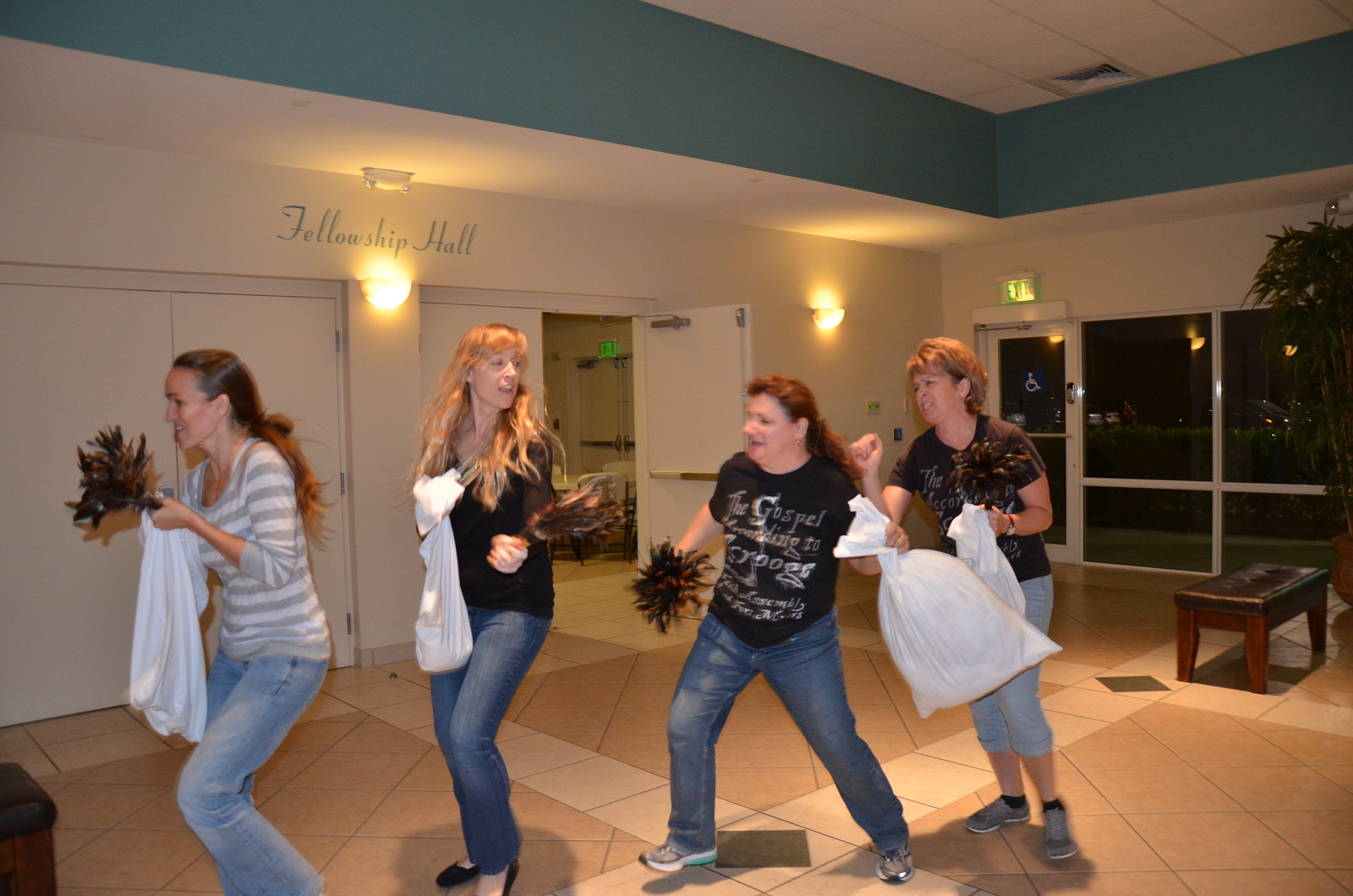This photograph captures an energetic scene featuring four women positioned diagonally from left to right, centered and more towards the left of the image. The setting appears to be the lobby of a hotel or possibly a church, suggested by the sign in the background that reads "Fellowship Hall," complete with white walls and teal accents at the top. The area is further illuminated by overhead white ceiling tiles.

From left to right, the first woman stands side-profile, holding a feather duster in one hand and a cloth in the other. She is dressed in a horizontally striped shirt (white and gray) and blue jeans, with long brunette hair tied in a ponytail that drapes past her shoulder. The second woman, clad in a black shirt and blue jeans, gazes towards the center of the photo at the woman to her right, clutching a similar feather duster and cloth, her long blonde hair flowing freely.

Next, the third woman is in mid-motion, perhaps dancing, with one foot lifted and weight shifted back. She carries a duster and what appears to be a pillowcase, dressed in a black shirt displaying some white and gold text (though obscured by wrinkles), blue jeans, and gray shoes. Her long brunette hair is tied back in a ponytail. The final woman on the right appears ready to join in the fun, also brandishing a duster and cloth, the other hand seemingly forming a fist. She has short blonde hair reaching her ears and wears a black shirt with similar white and gold text, blue jeans, and gray shoes.

The background reveals an emergency exit, a partially open double door, and another set of closed double doors. Further to the right, a green plant, along with a wooden and leather stool, can be seen. It appears to be nighttime outside, indicated by the view through tall windows.

The detailed tile floor is a blend of peach and cream hues with occasional diamond patterns, adding warmth to the setting. The women seem to be engaged in a lively activity, possibly a playful cleaning session or an impromptu dance, amidst an event or gathering, contributing to the spirited atmosphere in the Fellowship Hall.